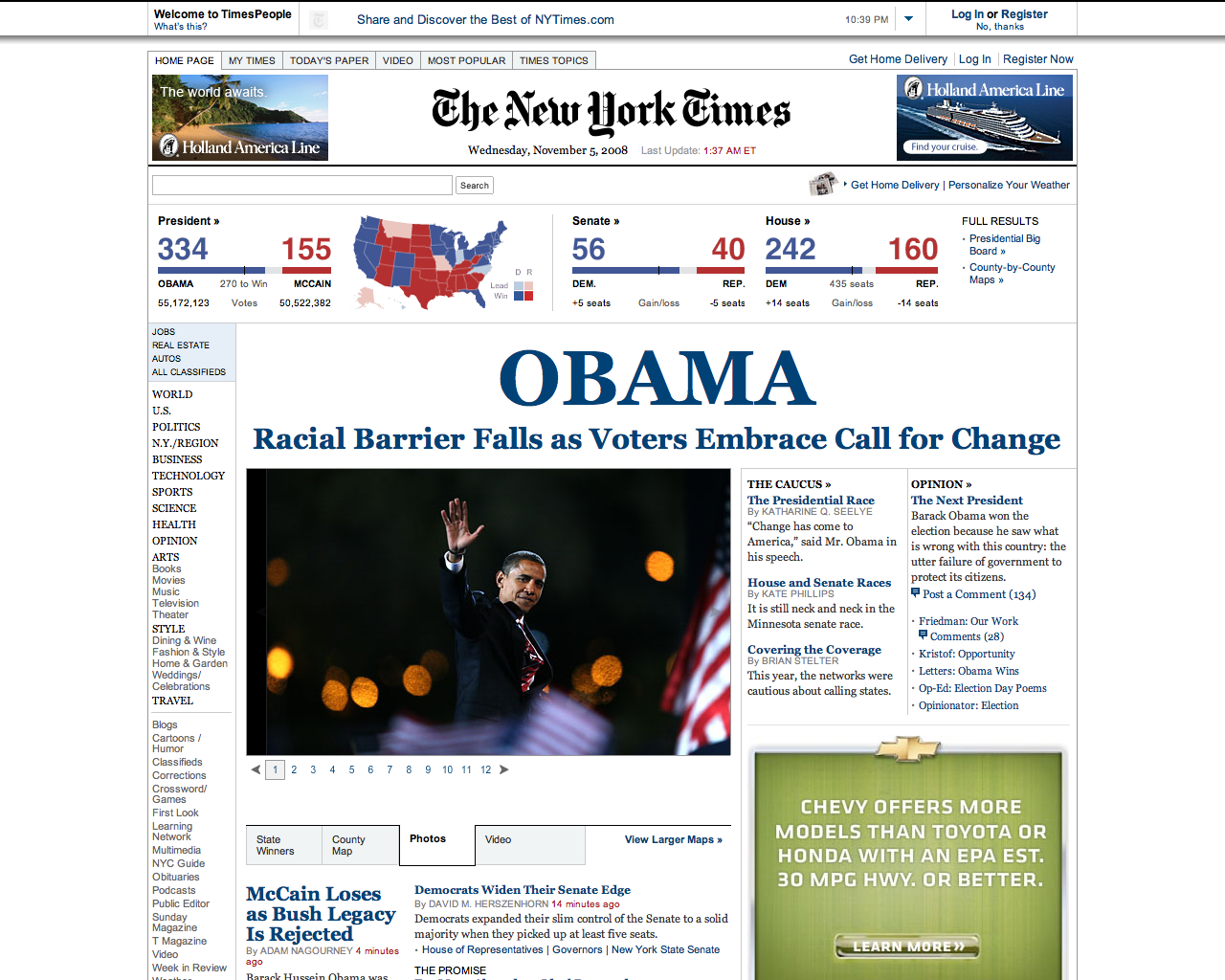This webpage screenshot features a comprehensive and detailed layout from the New York Times website. At the top-center of the page, the New York Times logo is prominently displayed in a dark black font with a traditional and elegant typeface. On the top-left, a friendly message reads, "Welcome to the Times, People," followed by "Share and Discover the Best of NYTimes.com." On the top-right, the digital clock shows a barely visible time, reading around 10 PM. Further right, there are options to "Log in" or "Register."

Flanking the New York Times banner are two vibrant advertisements for Holland America Line, showcasing picturesque beach and ocean scenes on one side and the cruise ship itself on the other. Below the logo, the date "Wednesday, November 5, 2008" and the last update time of "1:37 AM Eastern Time" are visible.

The navigation bar below offers six tabs: "Homepage," "New York Times," "Today's Paper," "Video," "Most Popular," and "Times Topics," with "Homepage" being highlighted. Additionally, on the right side of this section, three tabs offer options for "Get Home Delivery," "Log In," and "Register Now."

The dominant portion of the screen focuses on the historic election of President Barack Obama. The headline "Obama" is written in large blue font, with the subheader "Racial Barrier Falls as Voters Embrace Call for Change." Below, a striking photograph captures Barack Obama, a smiling African American man with short black hair, waving with his hand raised. He is dressed in a dark suit, paired with a red and white tie. The background of this image shows a blurred American flag, numerous small flags in the forefront, and a pitch-black backdrop lit with small yellow circles.

Above this featured image, election statistics are displayed with a map showing red states for John McCain and blue states for Barack Obama. Barack Obama secured 334 electoral votes with a final count of 55,172,123 votes, while John McCain garnered 155 electoral votes and 50,522,382 votes. The Senate race chart indicates 56 Democrats and 40 Republicans, and the House results show 242 Democrats to 160 Republicans. 

On the left, just beneath the headline “Obama,” a menu highlights categories including "Jobs," "Real Estate," "Autos," and "All Classifieds," along with other sections like "Style," "Fashion," "Opinion," "Cartoons," and "Obituaries."

Below Barack Obama's photo, an article titled, "McCain Loses as Bush Legacy is Rejected" by Adam Nagourney is featured. To the right, there are several articles including the headline "The Caucus" with three articles beneath it and "Opinion" with one article and several clickable tabs like "Letters" and "Obama Wins." Finally, there is an ad for Chevy on the far right side of the page.